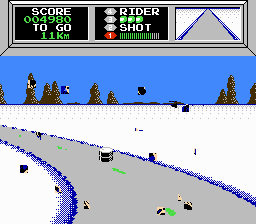This image is a pixelated screenshot of an old racing video game, reminiscent of graphics from Microsoft Paint. At the top, a blue sky stretches across the screen, adorned with some cedar trees peeking out from behind a high white wall that lines the racing track. The track itself, resembling the layout from the classic game Pole Position, winds through the middle of the image and is accompanied by small, brownish squares that likely represent pixelated racing characters or obstacles. The road appears gray, with blips that imply the presence of other cars. The interface shows a score of 4980 and an indicator showing 11 kilometers remaining. The player displays include “4” for the rider, “3” as three green circles, “2” labeled as shot, and “1” in red with numerous lines beside it. The scene is filled with green splotches, perhaps depicting grass or other track features, emphasizing the game's vintage and simplified visual style.